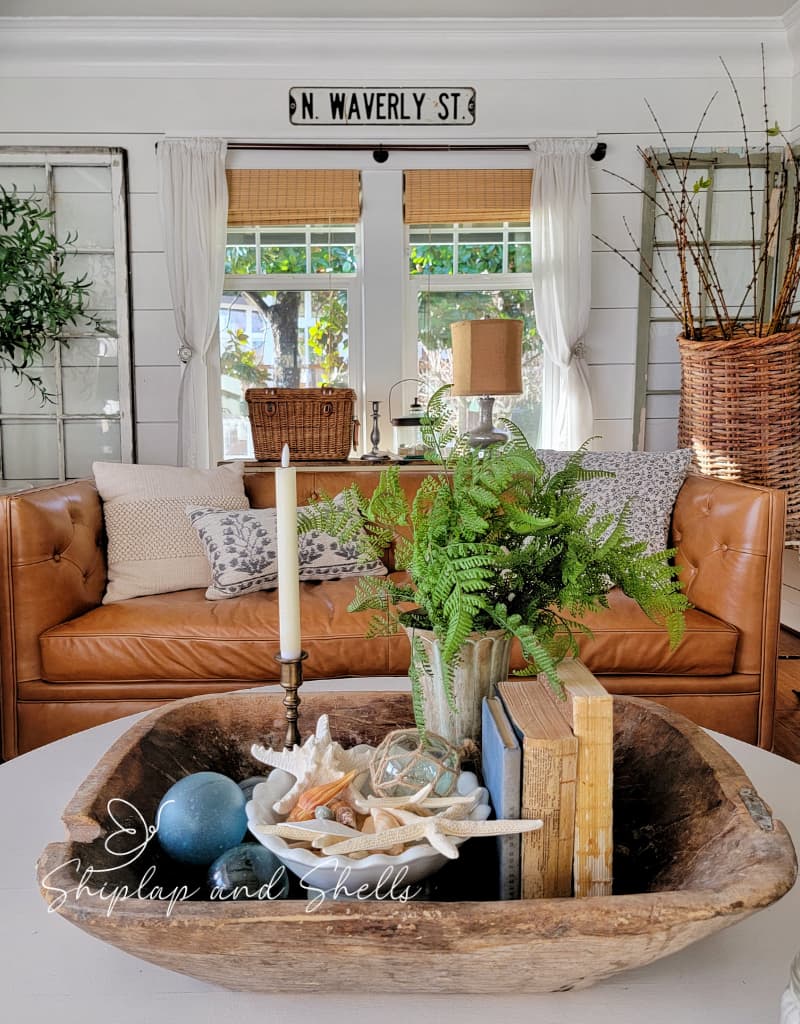This photograph captures a meticulously designed living room that could easily belong to a professionally curated interior. The focal point of the image is a circular or oval-shaped coffee table, showcasing a large rectangular wooden bowl with rounded corners. The bowl contains several old books to the right, a center vase filled with lush fern leaves, and a light blue scalloped-edged bowl holding starfish and a clear sphere at the front center. Additionally, there is a bronze candlestick with a white candle on the back left, accompanied by more clear or translucent spheres in the front left, adding an elegant touch to the display.

The backdrop features a medium brown leather couch adorned with pillows, including distinctive white ones with light blue or gray detailing, and one resembling a neck pillow. 

Behind the couch, the view extends to a pair of glass double doors framed with thin white drapes and topped with a brownish curtain. These doors allow a glimpse of the outdoor greenery, particularly thin brown trees with green foliage. There is also a coordinated aesthetic within the room, with white interior walls and various decorative items. 

A white sign reading "N. Waverly Street" in black text is prominently displayed above the doors, adding a personalized touch to the space. To the left of the couch, an array of decorative features includes baskets, dried twigs, and sticks. Clear windows lean against the wall purely for decor, with a hanging plant visible on the left and a large wicker basket filled with pussy willows on the floor to the right. Overall, the harmonious blend of rustic and natural elements, combined with comfortable furniture and thoughtful accessories, imparts a warmly inviting atmosphere to the living room.